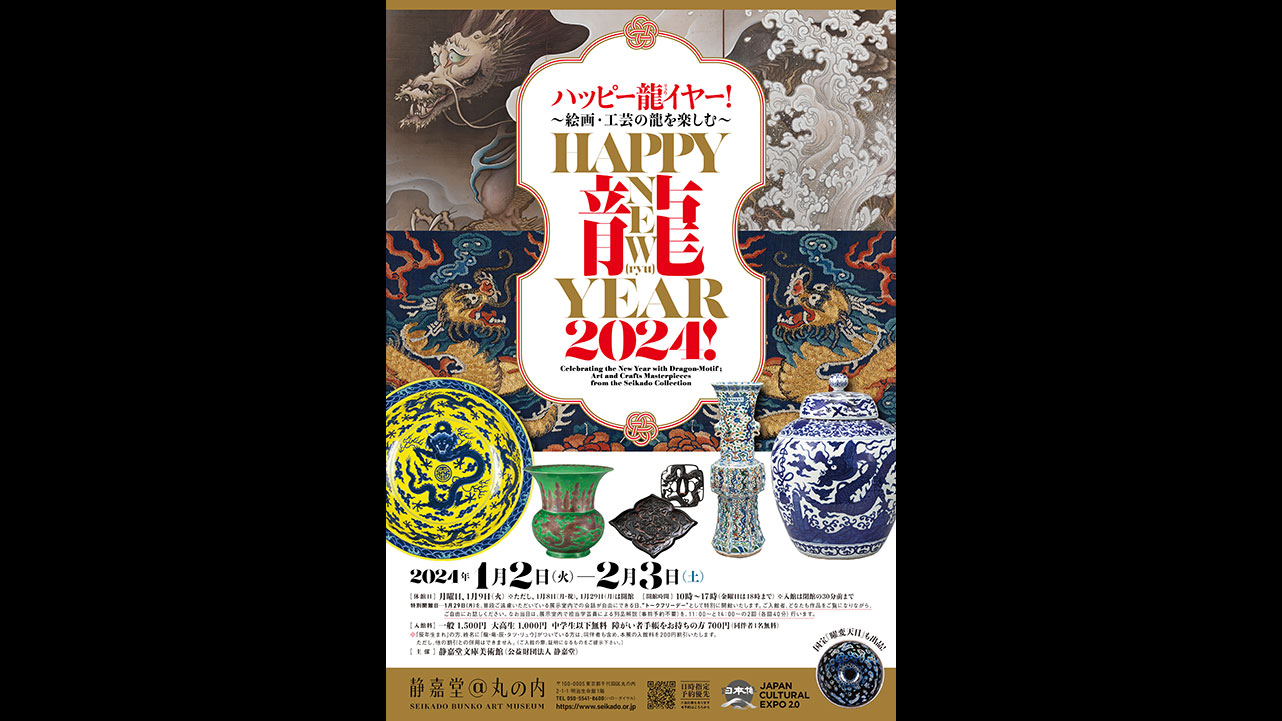This captivating poster, set against a black backdrop, announces a "Happy New Year 2024" sale, blending both Western and Asian elements. The "Happy New Year" text is stylishly presented, with "2024" standing out in bold red characters. Interspersed among this are Chinese (Mandarin) writings, lending an authentic cultural touch. The centerpiece of the poster features an array of elegant porcelain items: a stunning circular plate adorned with intricate yellow and blue patterns, a sophisticated green vase embellished with delicate pink designs, and a flat rectangular piece. Additionally, there's a beautifully crafted blue and white item that could either be a decanter or another vase, and an iconic blue and white lidded ginger jar. Below these exquisite items, more Chinese text likely details the specifics of the sale. The upper section's backdrop is enriched with traditional Asian drawings, including a prominent dragon motif, adding to the festive and cultural ambiance of the advertisement.